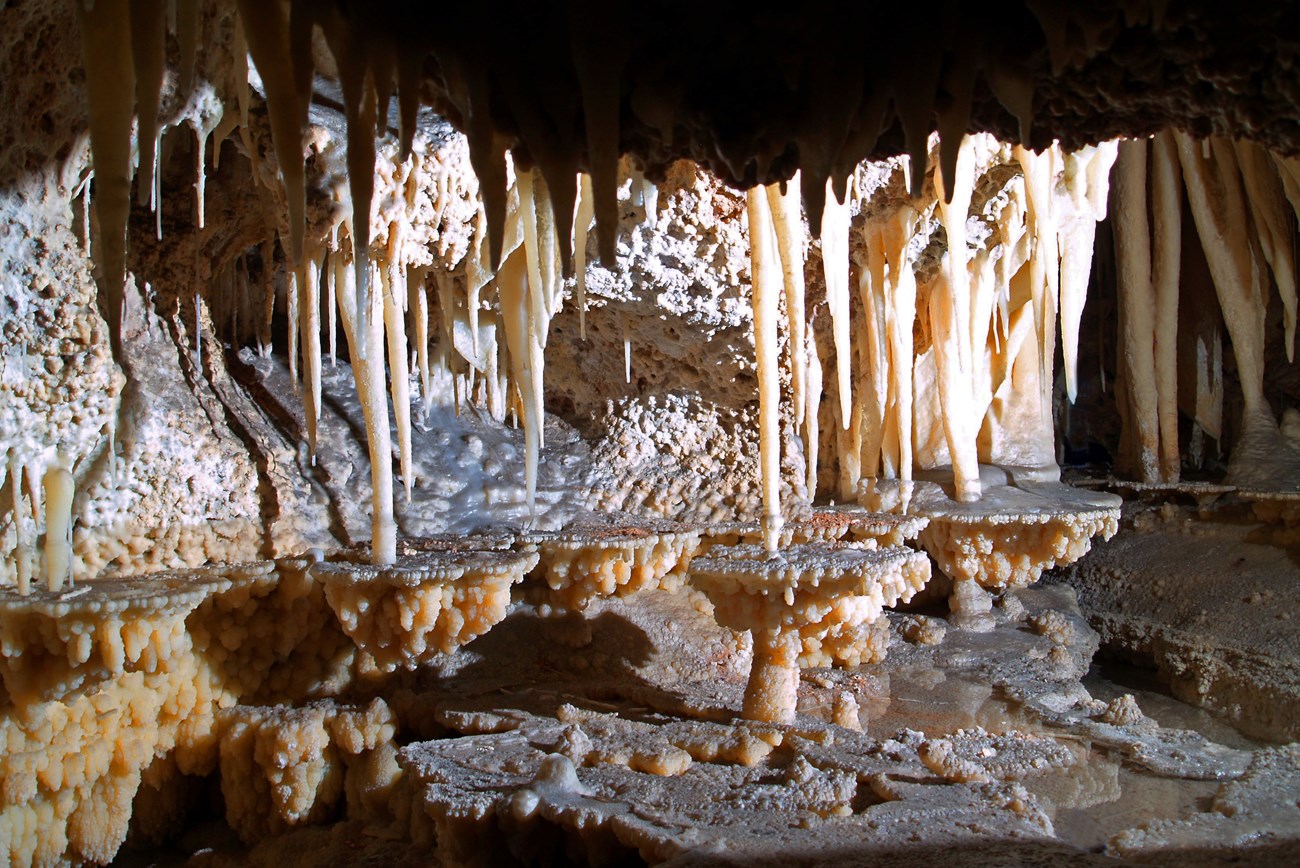This image captures a detailed, almost surreal photograph of the interior of a narrow cave. Dominating the scene are numerous stalactites, primarily white in color, hanging from the cave ceiling in various lengths and shapes. Some extend all the way down to the cave floor, creating almost mushroom-like structures with flat tops and lumpy, beige, and orange, bubbly bottoms. The cave walls and floor are rugged and irregular, covered in calcified deposits that give the formations a dripping, frozen liquid appearance. Light filters into the cave from an opening ahead, casting intriguing shadows and illuminating the reflective water pooled on the gray floor, accentuating the damp, mystical atmosphere of the cave.